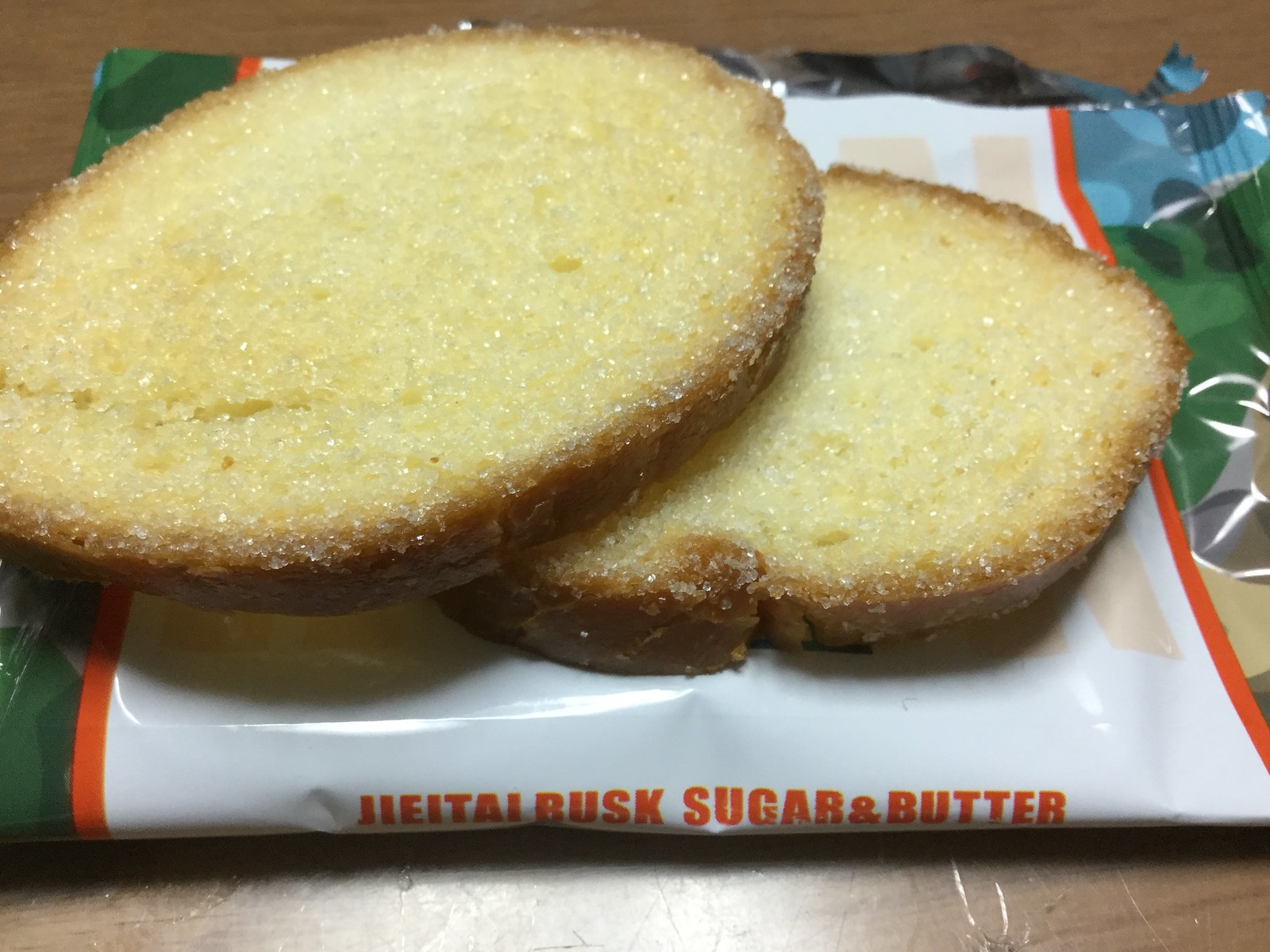This close-up image captures two slices of a distinctive sugar and butter bread sitting on an opened white wrapper with orange borders and orange text, which seems to read "HEITEL BUSK SUGAR AND BUTTER." The bread slices have a light yellow center and a nice brown crust, glistening with a sugar coating that gives them a sparkling appearance. The scene is set on a wooden table, adding a warm and rustic backdrop to the delectable treat. Overall, the bread appears to be slightly burnt, yet it looks delicious and inviting, making it a unique and relaxed visual.